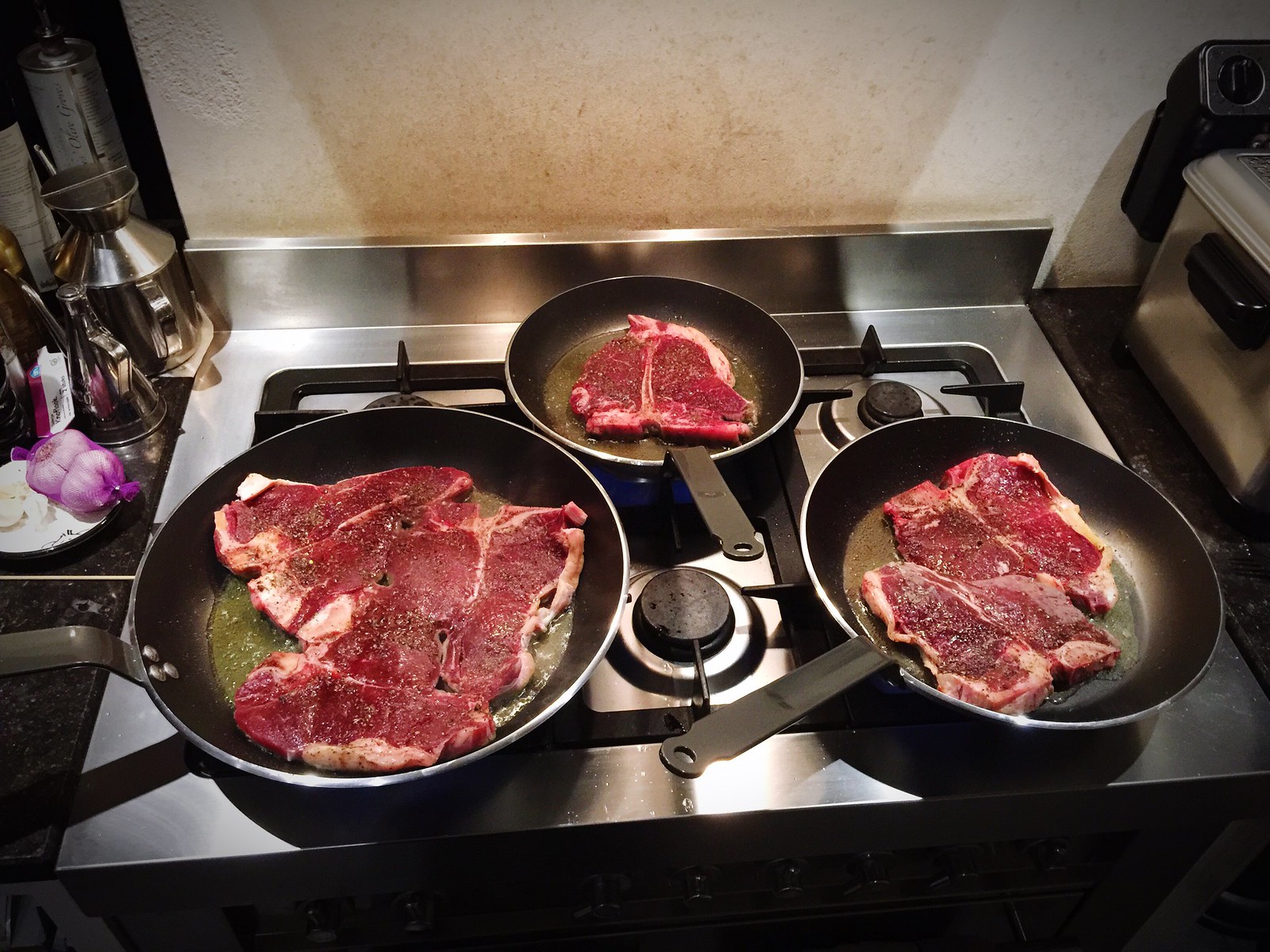This image depicts a stovetop with six gas burners, set against an off-colored white and slight brown wall. The sleek appliance features black burners, a silver metal lip at the back, and a black-and-silver aluminum base. Three frying pans dominate the scene: the largest pan is on the left, the next largest on the right, and the smallest in the middle near the backsplash. Each pan contains a red ribeye steak, outlined with white fat, and seasoned with black and white specks of salt and pepper. The steaks appear to be cooking in butter, with the burner under the smaller pan faintly glowing blue, indicating it's on. To the left of the stove, there are two silver oil cans and a light purple pepper, alongside a white plate with garlic wrapped in purple netting. The countertop is black marble and possibly a silver bread box is visible on the right side. The overall setup suggests either a high-end residential kitchen or a professional culinary environment.